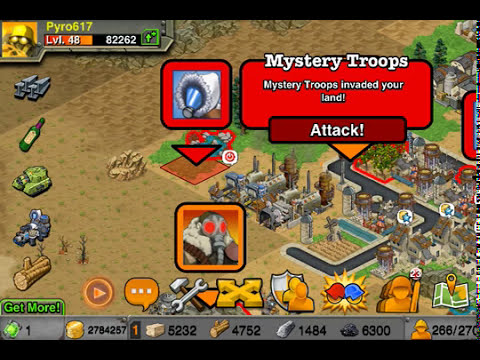This image is a screenshot from an older, somewhat rudimentary video game that appears to be military-themed. It shows a 3D aerial view of a landscape dominated by brown soil with patches of grass and industrial buildings, resembling a built-up town. The scene suggests a military engagement, as indicated by the red notification box with white text at the top stating, "Mystery Troops invaded your land, attack." Various icons are scattered on the screen, such as a crossed wrench and hammer symbol for building, and an icon representing an attack with two helmets clashing, surrounded by a yellow explosion. Below these icons are a map with a GPS symbol and numbers that likely indicate health, gold, or other resources. The top of the screen features a character named Pyro 617, detailed in yellow font alongside their level and score, displayed as "LVL 48" and "82262." The presence of characters, including one wearing a yellow suit and yellow hat, enhances the game's interactive elements, possibly allowing players to click on various bubbles to activate troops or engage in different actions.